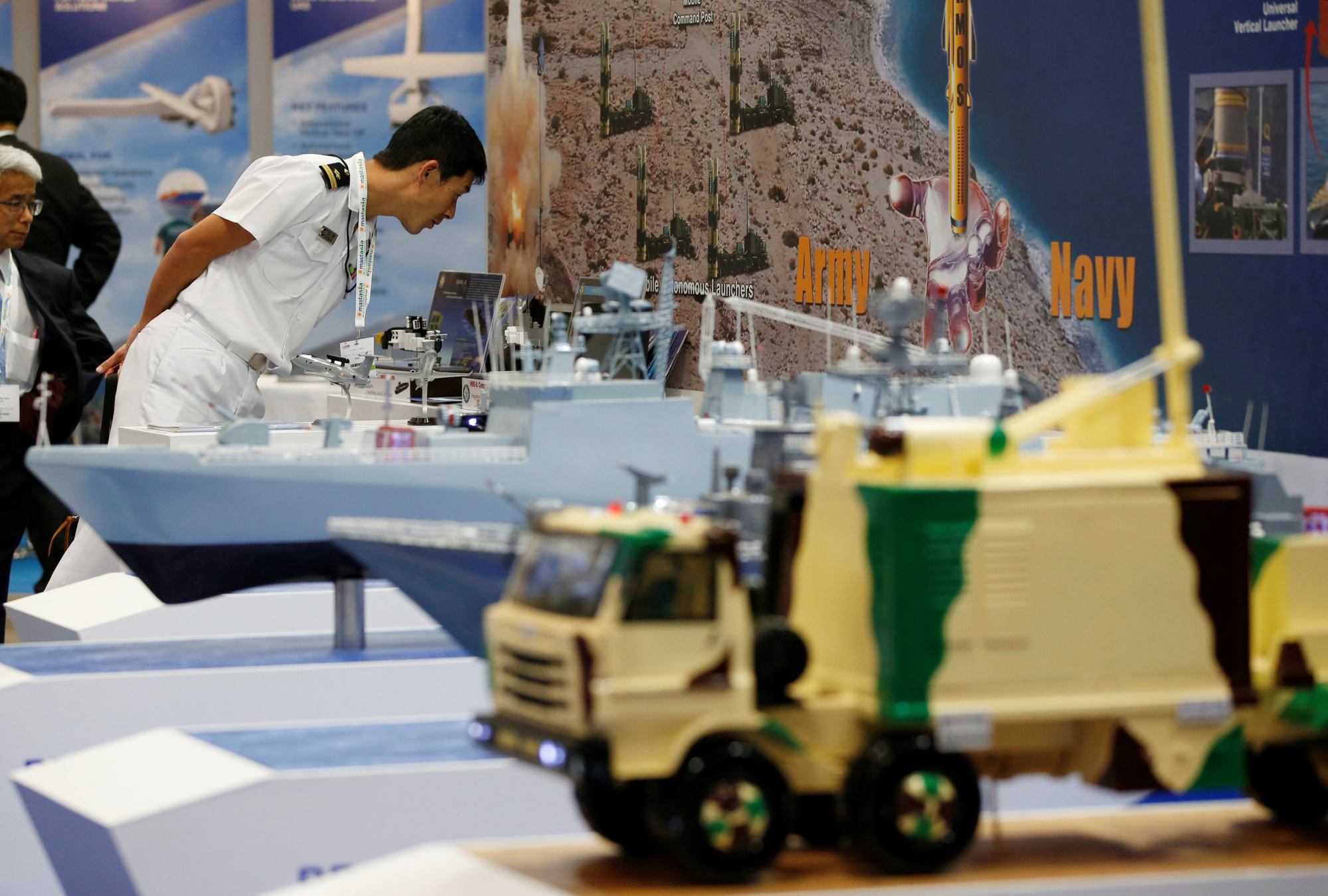The image depicts an indoor setting, likely a military museum or exhibit. The room is adorned with images and a backdrop featuring the words "Army" and "Navy" in bright orange, set against a striking landscape of desert and ocean. Multiple stands display scale models of military vehicles. In the foreground, an Army camouflage truck model is prominently featured. Behind it, there are several Navy vessel models. A man in a full white naval uniform is bent over a laptop or computer, seemingly engrossed in his task. A few other visitors can also be seen walking around, examining the various exhibits.